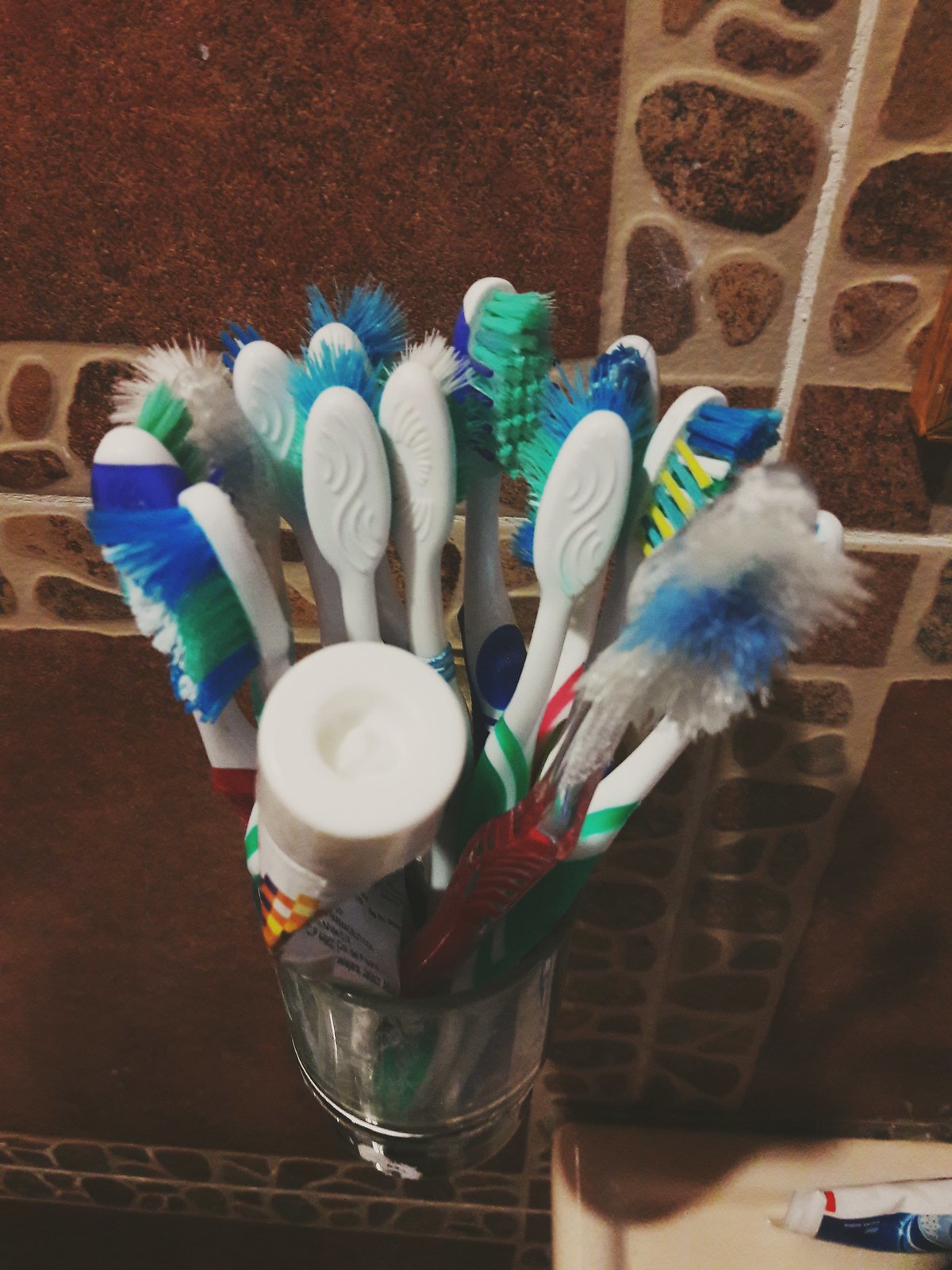The image captures a close-up of a shiny metal cup brimming with numerous heavily used toothbrushes and a tube of toothpaste with a white cap. The toothbrushes, varying in handle colors but uniformly sporting frayed and splayed bristles, signify that they are overdue for replacement. The metal cup is situated next to a sink and mounted against a distinctive wall composed of red, brown, and light brown tiles with a rocky design. In the foreground, there is also a glimpse of a porcelain toilet in the bottom right corner, which has an additional tube of toothpaste resting on its surface. The overall scene seems to evoke a sense of clutter and neglect, perhaps subtly commenting on the need for maintenance and renewal.